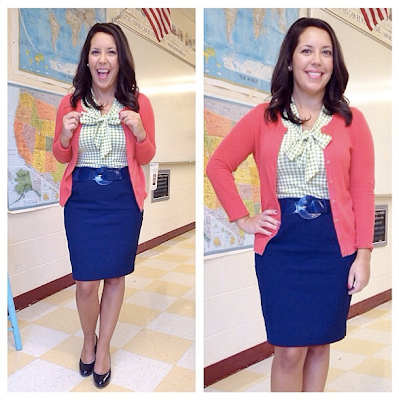The split view image features two photographs of the same woman, likely in a school classroom setting. She stands in front of a white cement block wall adorned with an American flag, two maps, a whiteboard, and a black sign with some writing on it. The woman, who might be a teacher, is dressed in a checkered red and white blouse with a ribbon, a pink unbuttoned cardigan, a shiny blue belt with a large buckle, a blue jean skirt, and either brown or dark-colored high-heeled shoes. In both images, she has brown hair and a big smile on her face. In the left panel, her arms are pulled in, while in the right panel, she poses with her right hand on her hip and her left arm down. The photographs also highlight her painted fingernails. The overall color palette includes royal blue, coral pink, white, beige, yellow, orange, red, pink, green, purple, and black.